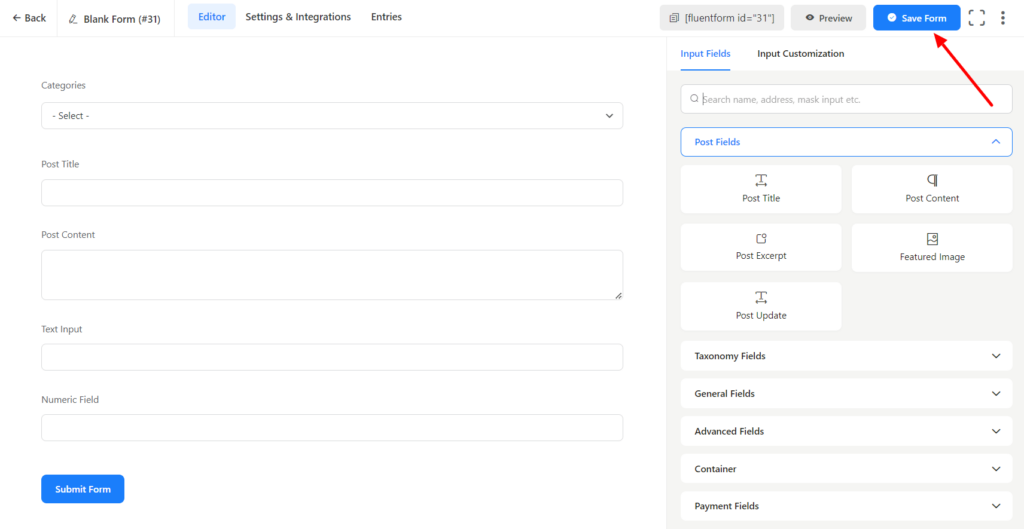The image displays a webpage with various interface elements designed for form editing. 

At the very top, a navigation bar features a left arrow icon for navigation, a blank input form, the number 31 enclosed in parentheses, and a pencil icon for editing. Below this, a blue-shaded box contains tabs labeled "Editor," "Settings and Integrations," and "Entries."

On the left side of the page, there are several rectangular boxes for inputting different kinds of information, ending with a blue "Submit" button. 

To the right, there are informational boxes; one reads "Fluent Form ID [31]" while another contains options labeled "Preview" and "Save Form," the latter highlighted in blue. A long, thin red arrow points upward to emphasize the "Save Form" button.

Below these elements, there are sections labeled "Input Fields," "Input Customization," and a search box, where "Input Fields" appears to be clickable. Another box labeled "Post Fields" also seems clickable and is accompanied by options such as "Post Title," "Post Content," "Post Excerpt," "Featured Image," and "Post Update." There are five additional fields with various other options.